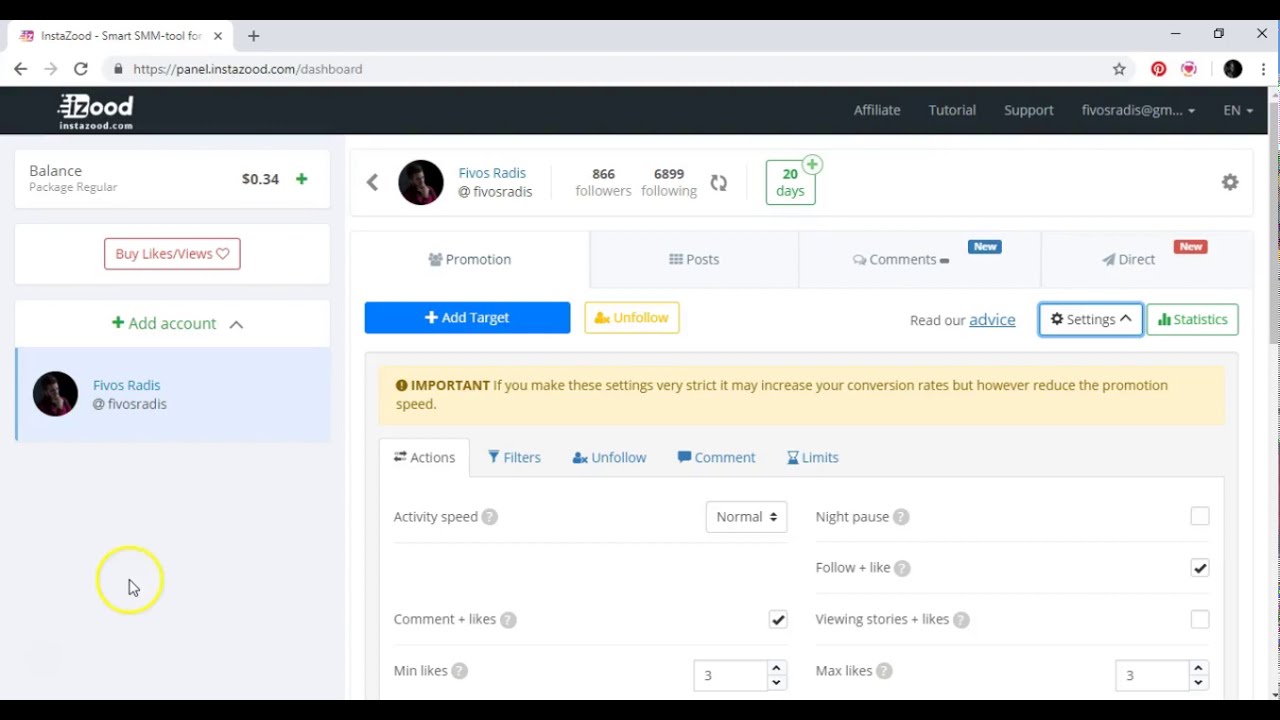This is a detailed screenshot of a web browser displaying a single active tab for the URL "panel.instazood.com/dashboard". The page belongs to the social media management tool "iZood". The top band of the screen features typical web browser navigation elements including back and forward buttons, a reload button, and the address bar, which clearly shows "panel.instazood.com". The dashboard prominently displays multiple feature tabs like Activity, Speed, Comments, Likes, Filters, and more, providing comprehensive metrics and functionalities for social media enhancement.

On the right-hand corner of the dashboard, there are options labeled "Affiliate", "Tutorial", and "Support", along with a language selection drop-down, all presented in white text. The upper portion of the site includes a section titled "Balance" showing 34 cents, and options to "Add Account". The account details for "Fivos Radice" are visible, listing 866 followers and 6,899 following. Additionally, there are tabs such as Promotion, Post, Comment, and Directs, indicating various tools available for boosting social media engagement. The page features a minimalist design with a white background interspersed with graphical columns and relevant textual information for managing social media accounts.